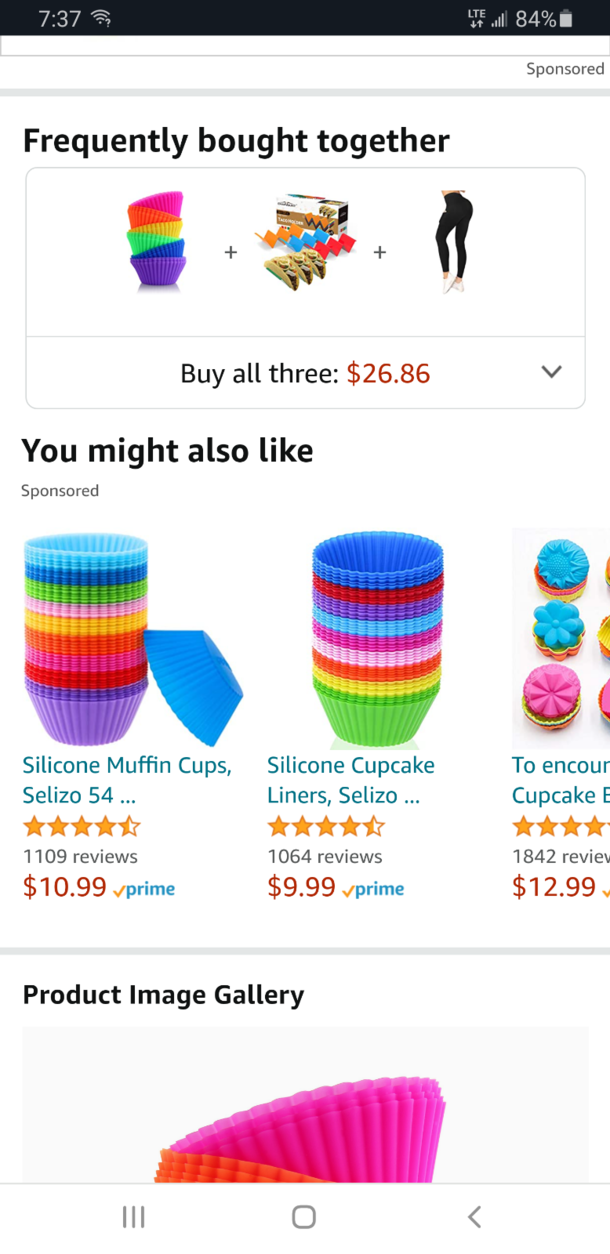Screenshot of an Amazon product page displaying a "Frequently Bought Together" section. Featured products include a set of cupcake liners, a zigzag-shaped taco holder, and a pair of leggings. Beneath these items, there is a combined price of $26.86 for purchasing all three. Further down the page, a "You Might Also Like" section appears, showcasing two additional sets of silicone cupcake liners. Below this section, there is a label indicating a "Product Image Gallery."